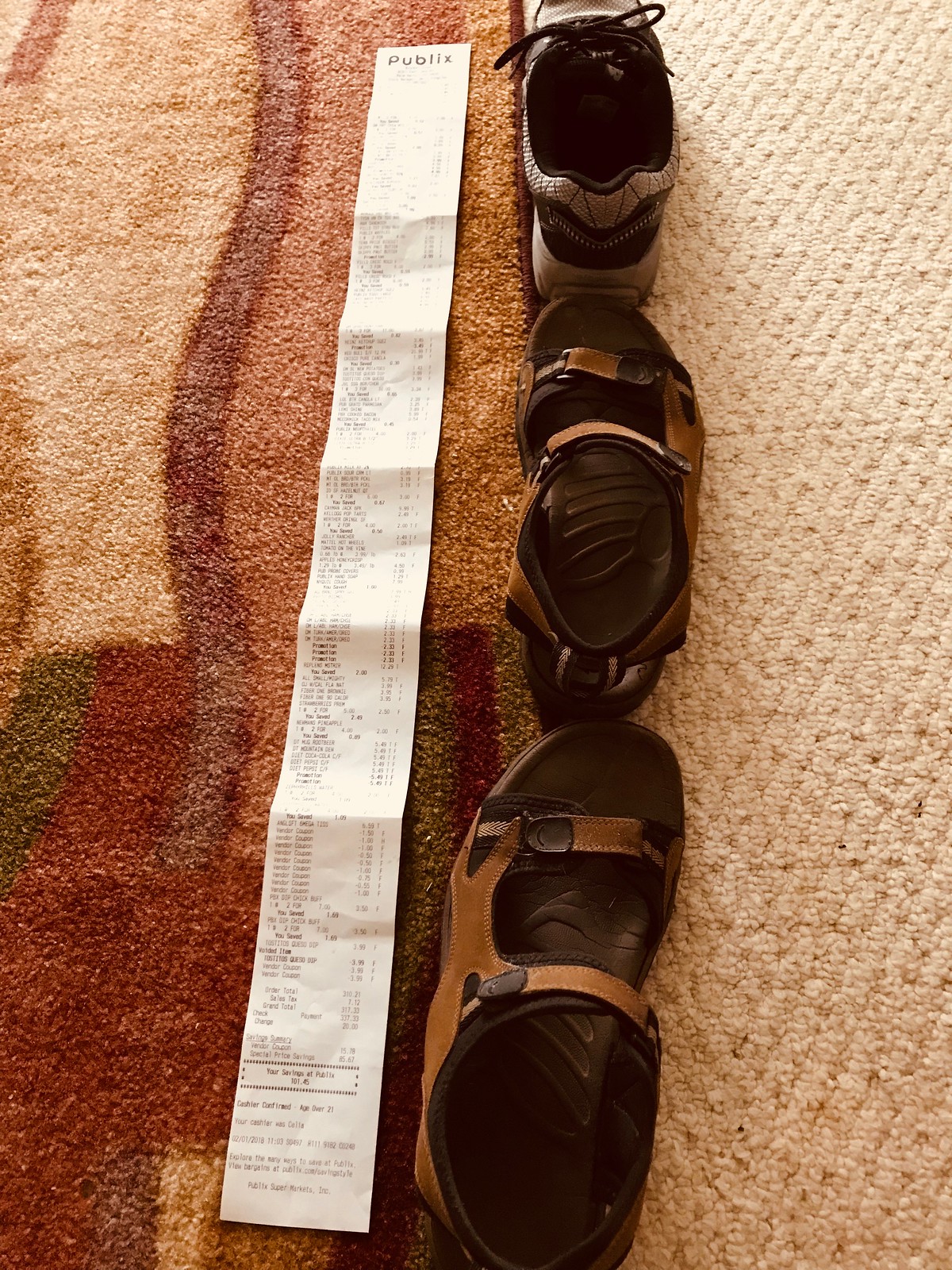This high-quality photograph, taken from a bird's eye view, captures a scene likely set in a room. The floor features a beige Berber carpet, partially covered by a red, brown, and tan rug. Laid out on the rug is an exceptionally long receipt from Publix, spanning the length of three men's shoes—estimated to be sizes 12 or 13. The three shoes are arranged in a vertical line, top to bottom: a gray sneaker, a brown right sandal, and a brown left sandal. The white receipt, possibly over four feet long and bearing the Publix logo at the top, visually aligns with the shoes. It's filled with numerous purchased items, suggesting a total expenditure between $200 and $300. The composition emphasizes both the considerable length of the receipt and the contrasting textures and colors of the shoes, rug, and carpeting.